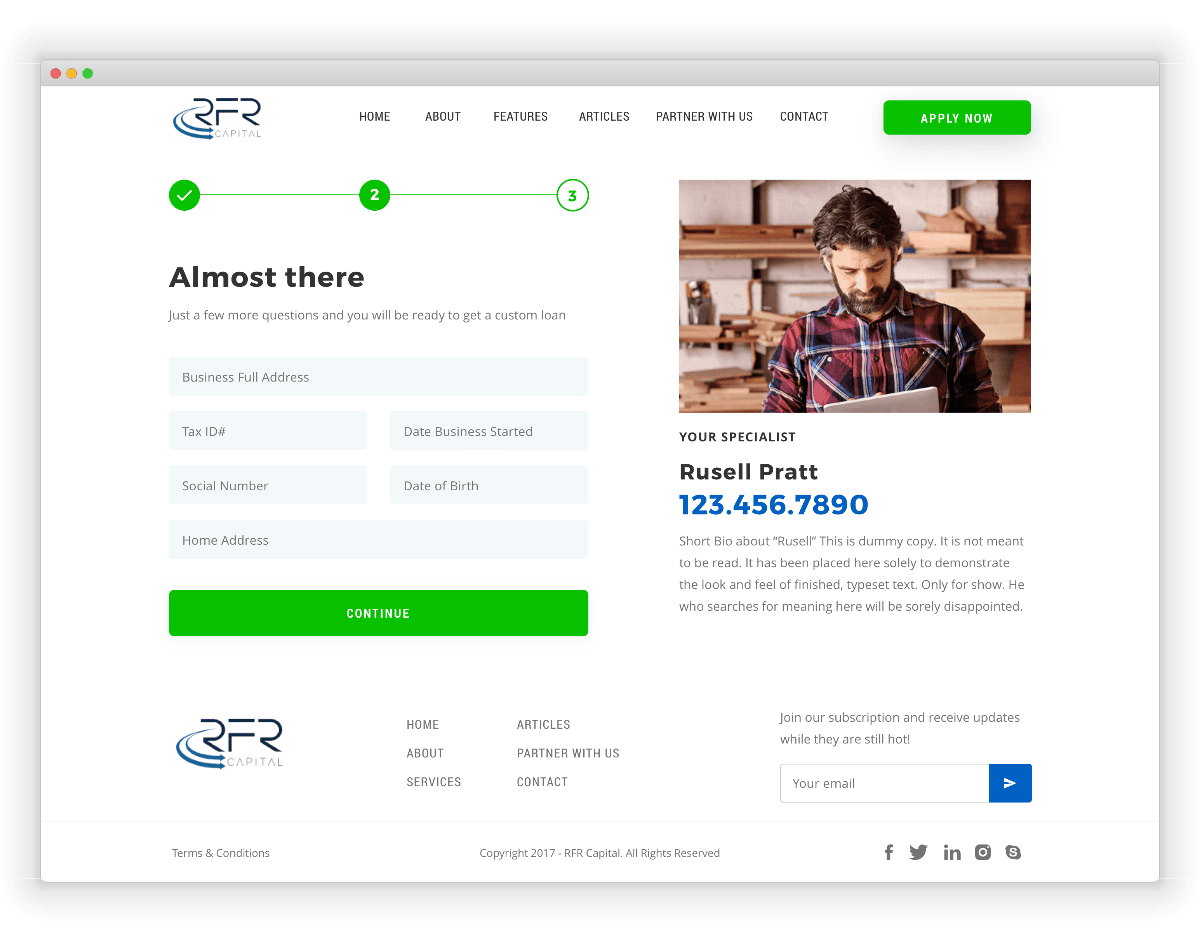The image is a screenshot from the RFR Capital website. The top of the screen features a gray bar spanning the width of the page, displaying three colored circles (blue, red, yellow, and green) aligned horizontally. Below the bar, the text "RFR" appears in black, with "Capital" in gray next to it. Intersecting this text are two blue arrows: one originating from the open part of the "R" on the left, curving outwards before swinging back into the word "Capital."

To the right of the RFR Capital logo is a navigation menu with the options: "Home," "About," "Features," "Articles," "Partner with Us," and "Contact," all in black capital letters on a white background. Adjacent to this menu is a green "Apply Now" button with white text.

Below this section is a series of green and white circles linked by green lines, leading from a white checkmark in a green circle, to a white "2" in a green circle, and finally to a green "3" in an outlined green circle. The text "Almost there," in bold black font, is followed by a message: "Just a few more questions and you will be ready to get a custom loan," in regular black text.

Further down is a light blue box labeled "Business Full Address." Beneath this are smaller boxes for "Tax ID Number" and "Date Business Started." Additional fields include "Social Security Number," "Date of Birth," and "Home Address." At the bottom of these input fields is a long green "Continue" button with white text.

In the top right corner, there is a photo of a man with a beard and mustache, dark brown hair with some gray at his temples, wearing a red plaid flannel shirt. He is looking down at either papers or a tablet, in front of a backdrop of wooden shelves. Below the image is the text "Your Specialist," with the name "Russell Pratt" in bold. A bold blue phone number, "123.456.7890," is listed, followed by gray text stating, "This is a dummy copy. It is not meant to be read. It has been placed here solely to demonstrate the look and feel of finished typeset text, only for show. He who searches for meaning here will be sorely disappointed."

In the bottom left corner of the screen is another RFR Capital icon, next to a footer menu with the same navigation options: "Home," "About," "Services," "Articles," "Partner With Us," and "Contact" in gray capital letters. To the far right, there's a section inviting users to "Join Our Subscription and Receive Updates While They Are Still Hot!" featuring a field for "Your Email" and a blue square with a white right-pointing arrow.

At the very bottom of the page are the terms and conditions in black text, "Copyright 2017-RFR Capital, All Rights Reserved," followed by social media icons for Facebook, Twitter, LinkedIn, Instagram, and Skype.